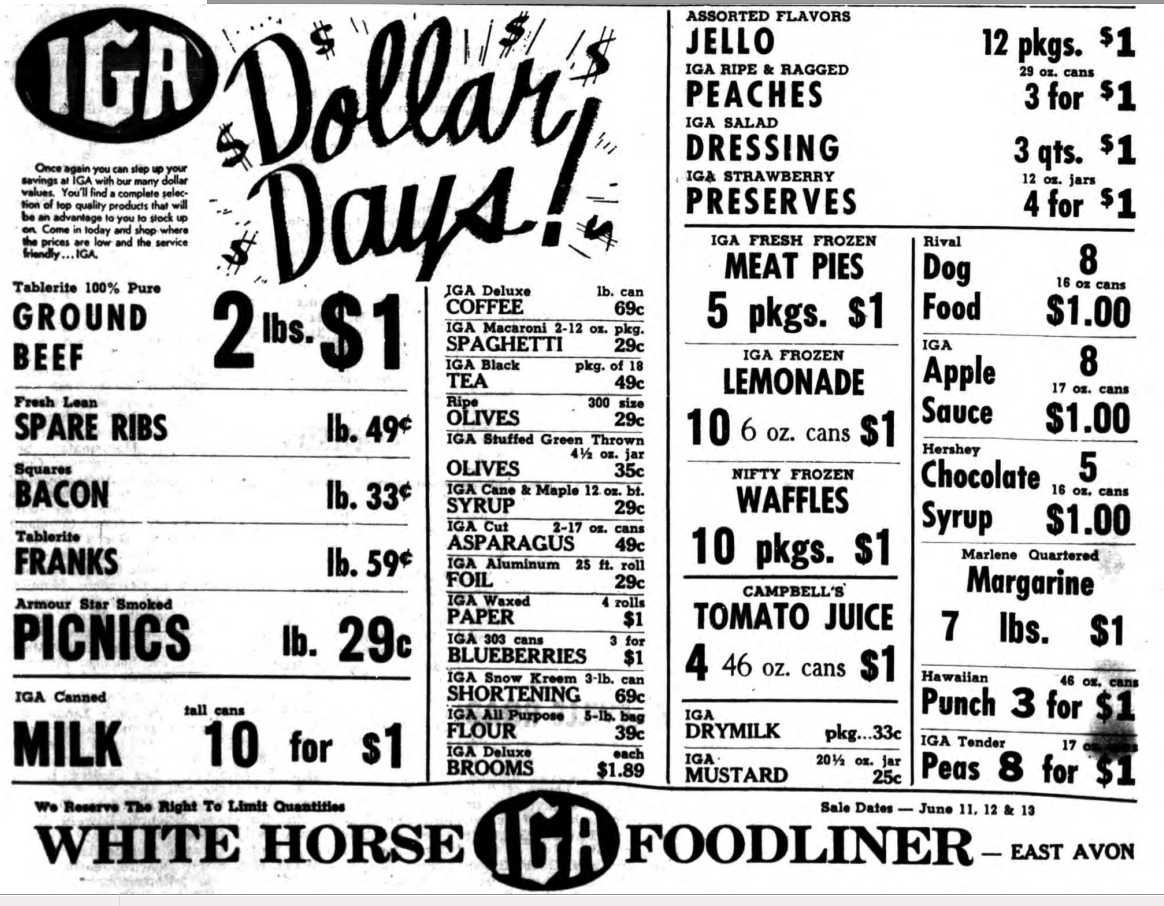This black-and-white grocery store flyer from a bygone era advertises dollar days specials from the White Horse Food Liner on East Avon Street. The flyer prominently features the IGA logo, a black oval with white letters, in the upper left corner. Immediately to the right, bold text exclaims "Dollar Days!" with an exclamation mark. Below the logo, there's some small, unreadable black text. The page is divided by a vertical black line running down the middle, creating two main columns.

In the left column, various meats and dairy products are promoted, including ground beef (two pounds for a dollar), spare ribs, bacon, franks, smoked picnic salad, and milk. The right column, split again into two smaller columns, lists more items with prices in smaller text. Notable deals here include coffee (one-pound can for 69 cents), spaghetti, tea, olives, syrup, asparagus, aluminum foil, wax paper, blueberries, flour, and brooms. The top right section of this column highlights specials like assorted flavor Jell-O (12 packages for a dollar), peaches, dressing, and preserves.

The flyer specifies that all these items range in price from 33 cents to a dollar, suggesting it was printed at least 30-40 years ago. Signifying its age further, the sales dates are noted as June 11, 12, and 13. Finally, the bottom of the flyer states, "White Horse IGA Food Liner - East Avon" with a disclaimer above on the right-hand side reserving the right to limit quantities.